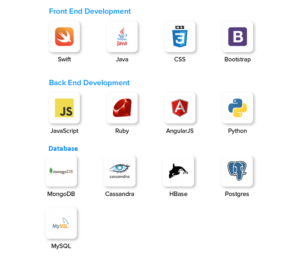The image showcases a neatly organized grid of square icons representing various computer programs and programming languages, specifically targeted towards different stages of development. The background is pure white, seamlessly blending into the image’s prolific layout. 

At the top, the title "Front End Development" is displayed in blue font. Below this title, there are four square-shaped icons with rounded corners and subtle drop shadows on the right and bottom edges. These icons represent:
- Swift: Featuring its signature logo.
- Java: Displaying its recognizable coffee cup emblem.
- CSS: With its familiar blue square and CSS3 insignia.
- Bootstrap: Showcasing a purple square within the white icon, containing a white "B".

The next section is titled "Back End Development" and consists of four more square icons, each denoting different programming languages and frameworks:
- JavaScript: Highlighting its iconic yellow background and "JS" logo.
- Ruby: Featuring its distinctive gemstone logo.
- AngularJS: Depicted with its angular shape and red background.
- Python: Displaying the intertwined yellow and blue snake icon.

The final section is labeled "Database" and includes icons for various database management tools:
- MongoDB
- Cassandra
- HBase
- PostgreSQL (noted as Pastgres)
- MySQL

Each icon is designed to visually represent the respective program it stands for. Collectively, these icons symbolize a comprehensive toolkit for front-end, back-end development and database management, suggesting that the image might serve as an interface where users can click on each icon to access the corresponding program.